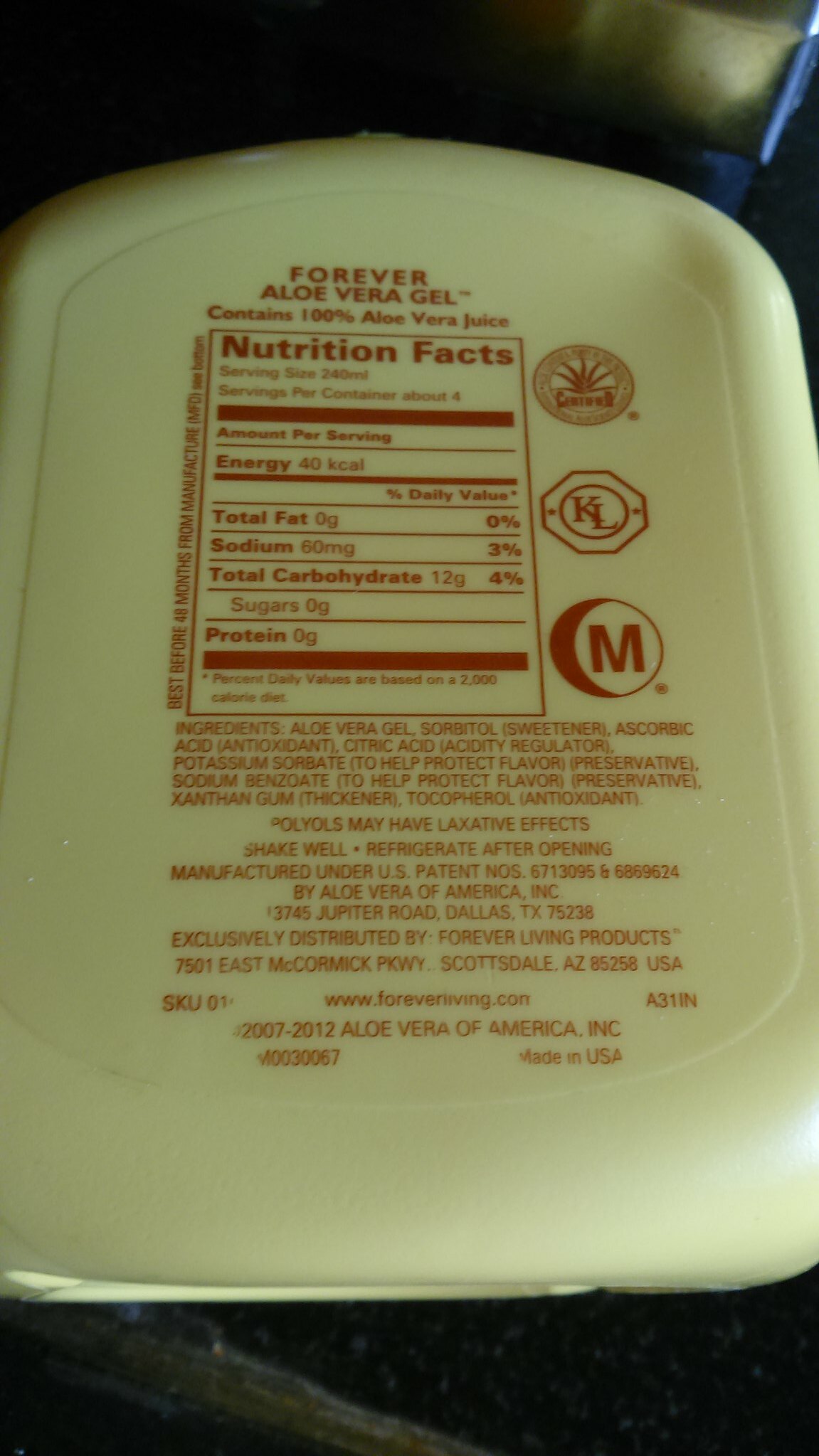The image depicts a color photograph of a container labeled "Forever Aloe Vera Gel," which prominently features red text on its off-white, opaque plastic surface. The container boasts that it contains 100% aloe vera juice. At the top of the label, "Forever Aloe Vera Gel" is written in small letters. Below this, there is a red-bordered rectangle housing the Nutrition Facts, detailing serving size (240 milliliters), servings per container (about 4), and nutritional content: 40 kcal, 0 grams total fat, 60 milligrams sodium, 12 grams total carbohydrates, 0 grams sugar, 0 grams protein. The label notes that percent daily values are based on a 2,000 calorie diet. Details also include a best-before period of 48 months from the manufacturer and an ingredients list specifying aloe vera gel, sorbitol sweetener, ascorbic acid antioxidant, citric acid acidity regulator, potassium sorbate and sodium benzoate as preservatives, xanthan gum thickener, and tocopherol antioxidant. It cautions that polyols may have laxative effects, instructs to shake well and refrigerate after opening. The label also mentions that the product is manufactured under U.S. patents by Aloe Vera of America Incorporated and is exclusively distributed by Forever Living Products, along with addresses and a website, www.foreverliving.com. To the right of the Nutrition Facts, there are three logos indicating various approvals, although their specific significance is unclear.